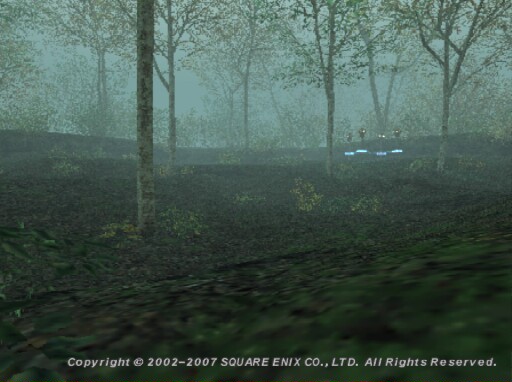This image captures a lush forest scene from the video game, Final Fantasy XI Online, specifically set in the Balafu Thickets within the Treasures of Aht Urhgan region. The viewpoint appears to be from the ground looking upwards. The foreground showcases green grass with some bushes and shaded areas. On the left side, a large tree trunk extends upward, partially cutting off the top of the frame. The middle section is filled with birch trees stretching across the skyline from left to right, with patches of blue sky peeking through. Just right of the central tree, another tree stands with visible branches and leaves. Further to the right, another tree is closer in view with dense branching. Between two trees on the far right, glowing eyes of indistinct small animals can be seen lurking. The bottom right corner features four pillars with rounded tops and blue bands encircling their middles. The image is slightly foggy, and the text at the bottom reads "Copyright 2002-2007 Square Enix Co., Ltd. All Rights Reserved." The sky in the scene is described as a steel gray, hinting at an overcast atmosphere.